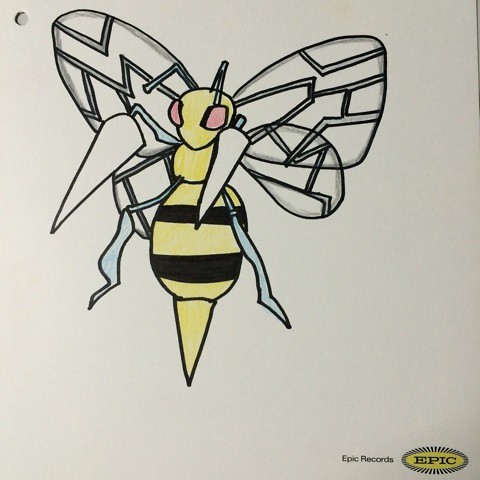This is a detailed sketch of a bee, resembling the Pokemon character Beedrill, drawn on khaki or tan paper with a hole punched in the top left corner. The bee is positioned slightly left of center, leaving more blank space on the right. It features red eyes and small antennae near its head. The bee's body is yellow with the classic black stripes and a pointed yellow stinger. Its legs and arms are blue, and it has sharp claw-like pincers. The wings are depicted with structural lines, appearing almost filamental. The bee seems poised for battle with an aggressive stance. The drawing appears to be traced or outlined with a thick black pen or thin marker, and colored in with blue, yellow, red markers, and possibly pencil. In the bottom right corner, the text "Epic Records" appears within a yellow circle, which has lines radiating from it like a sunburst.